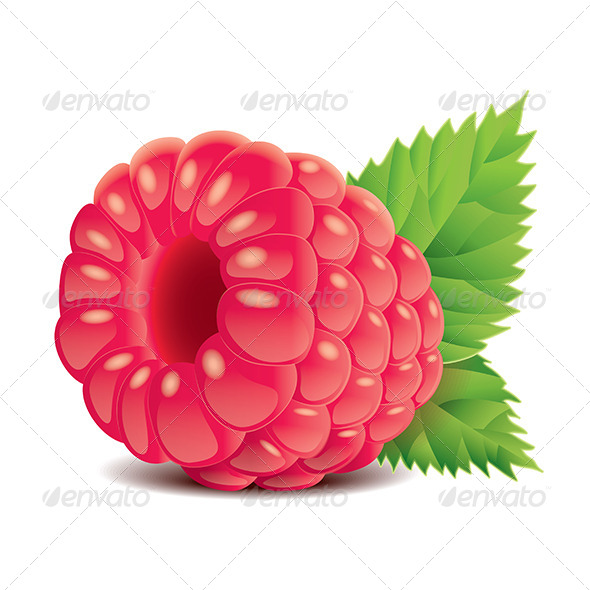The image is a highly detailed illustration of a single red raspberry, depicted with a vibrant reddish-pink body and a bright green stem and leaves at the top. The raspberry is positioned on a white background, with its hole facing the front - indicative of where it was picked from the plant. The fruit’s surface features detailed shading and subtle yellowish glints, giving it a shiny, ripe appearance. Each leaf on the stem is meticulously drawn, showcasing pronounced points and visible veins. A faint watermark reading "Envato" with a logo is present throughout the image. The watermark is accompanied by angled lines forming a subtle square grid pattern at the top of the image.